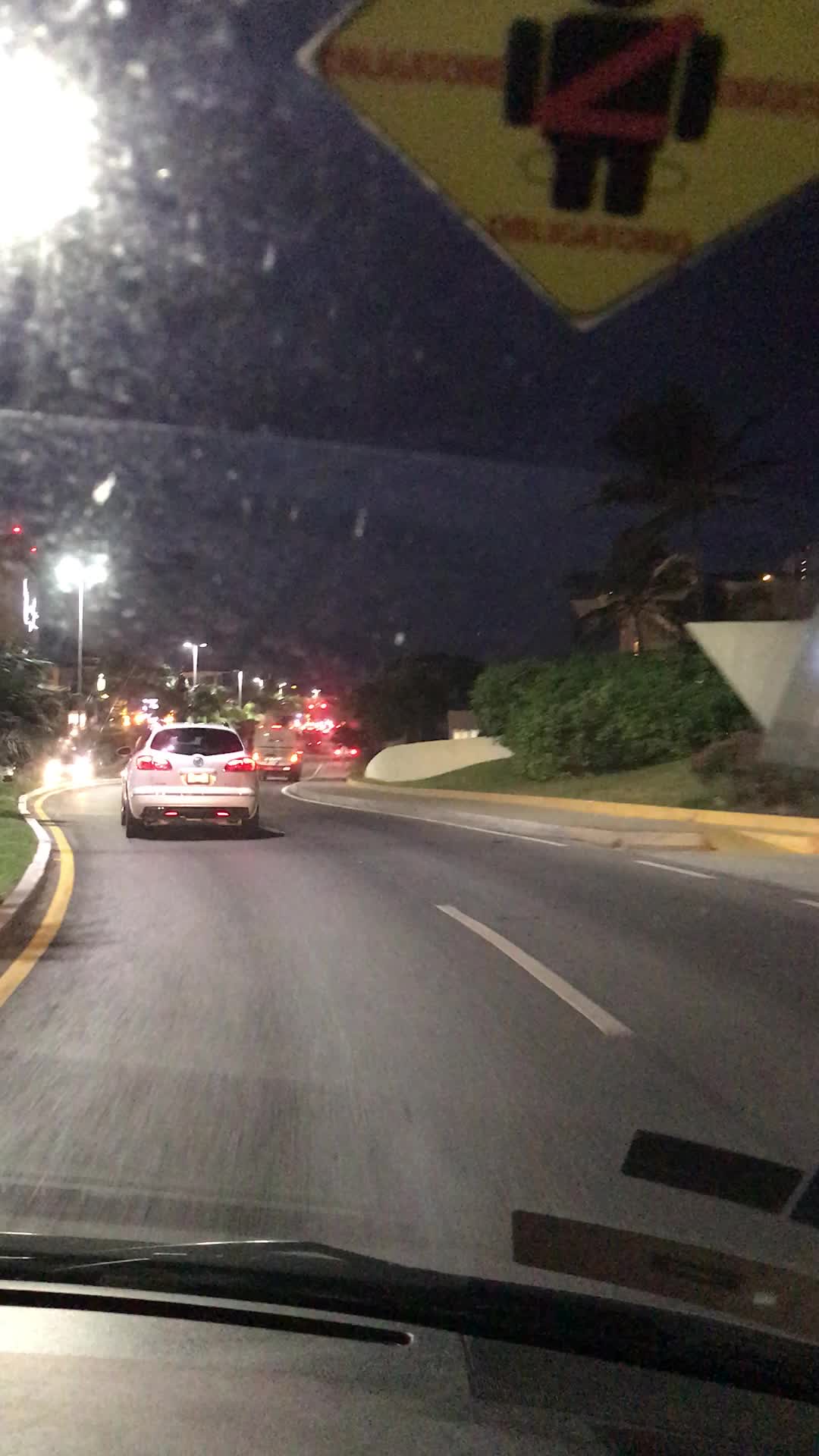A nighttime photograph captures the view from the passenger seat of a car, looking through a somewhat dirty windshield. The image depicts a curvy, two-lane road with yellow borders ahead. Several cars, including a white hatchback or crossover SUV directly in front, are visible, their red taillights bright against the dark surroundings. On the right side of the image, dense shrubs and brush can be seen, along with a large, dark tree that stretches over the road, partially obscuring the upper half of the picture. The car's black and gray dashboard is visible at the bottom, and a diamond-shaped yellow sign with an android figure wearing a red seatbelt hangs in the upper right corner of the windshield, though the text on it is not legible. The windshield's glare and the blurry light near the top left corner add to the overall obscure feeling of the image, making it unclear as to the photograph's intended subject or significance.